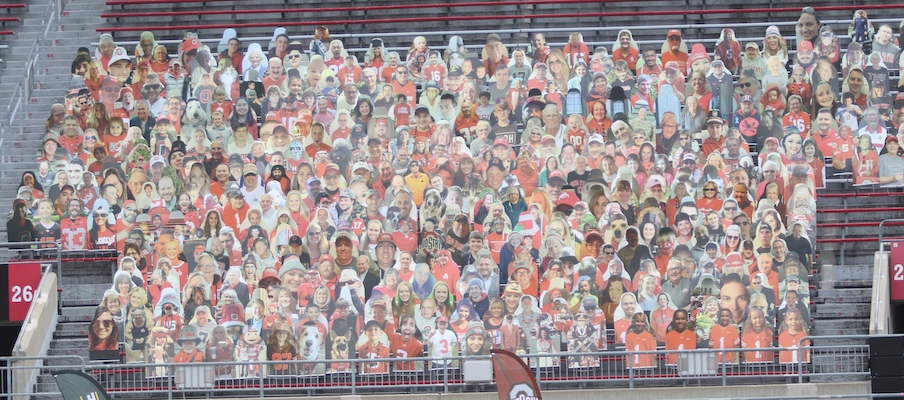The image displays a detailed scene of an Ohio State University football stadium during the COVID-19 lockdown. The focus is on the stands, which are heavily populated with cardboard cutouts of fans to simulate a real audience. These cutouts, which include a mix of people and pets, create the illusion of a packed stadium. Notably, several cutouts in the front right wear Ohio State jerseys marked with the number one. A prominent red banner with the number 26 hangs on the left side above a portal leading down to the playing field. The stands feature red seats, concrete stairs, and chrome handrails, giving the setting an authentic sports venue atmosphere. In the foreground, there's also a flag adorned with Ohio State's logo, emphasizing the collegiate football context of the scene.